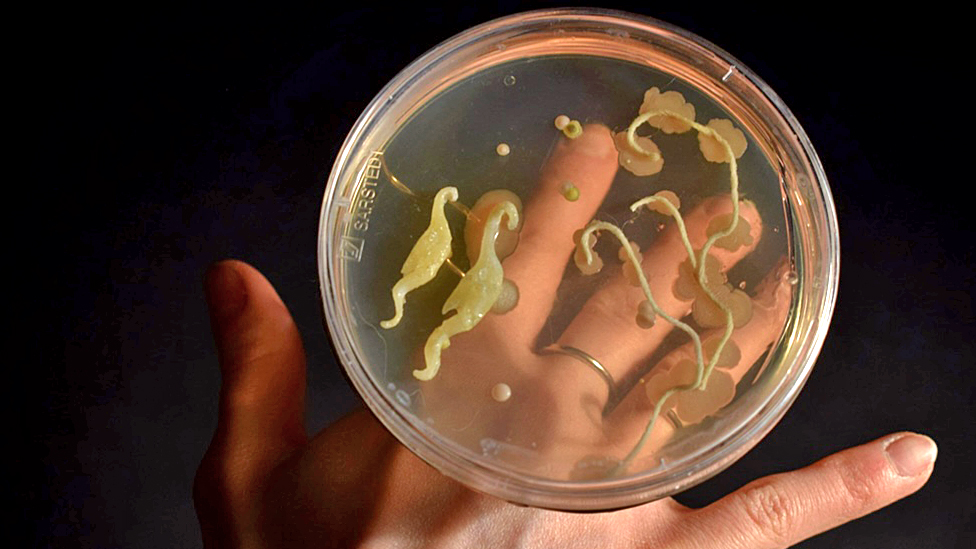The image features a transparent petri dish resting on the back of a live human hand, which is clearly visible beneath the dish. The hand, positioned flat against a dark black and blue background, has a slender metal ring on its middle finger. Inside the petri dish, there are intriguing and unusual biological substances. Two of these substances resemble miniature seahorses, while three others appear as thin string-like structures. The substances are yellowish and flesh-colored, adding to the mystery. Additionally, the petri dish bears the translucent lettering "S-A-R-S-T-E-D" on its left side, indicating the brand or type of the dish used in the experiment or culture process shown in the image.